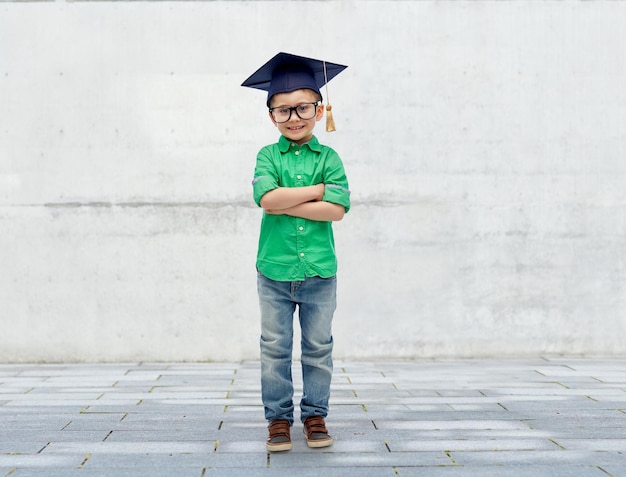In this outdoor daytime photograph, a young boy, possibly in preschool or kindergarten, stands confidently with his arms crossed over his chest. He is wearing a green, collared, long-sleeve shirt with the sleeves rolled up to just above his elbows, and he pairs it with blue jeans. His footwear consists of dark-colored velcro shoes in blue and brown. Atop his head is a dark blue graduation cap with a gold tassel gently hanging to the right side, giving him an endearing, nerdy vibe. The boy is smiling warmly at the camera, his eyes framed by glasses. He stands on a walkway made of gray rectangular tiles, with an off-white painted brick or concrete block wall in the background, adding a subtle contrast to the scene. Shadows or variations in tile shading play across the ground, adding depth to the image.